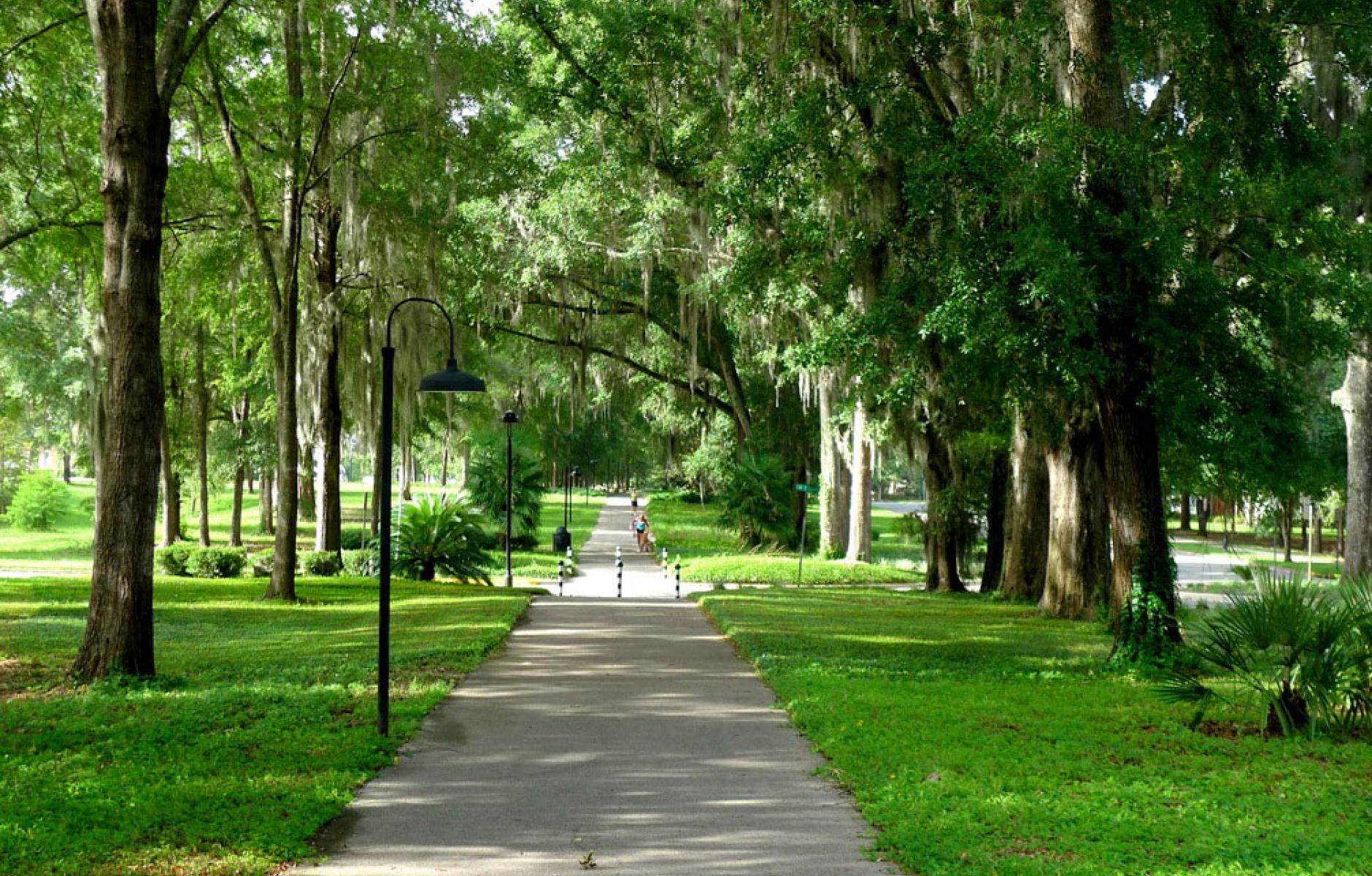The image showcases a scenic park featuring a well-maintained, gray cement footpath that stretches from the bottom center of the frame and disappears into the distance. The path, bordered on both sides by lush, vibrant green grass and tall trees, creates a canopy overhead. The trees, some draped with Spanish moss and possibly suggestive of a southern location, add to the park's serene atmosphere. Along the left side of the path, black street lights hang to provide illumination at night. Halfway up the path, three white poles with black stripes stand in a row, likely to prevent vehicles from entering and to caution pedestrians. The trail intersects with a street marked by a green street sign, though the name is not legible. In the distance, a few people can be seen walking, jogging, and walking a dog, adding a sense of life to the tranquil setting.